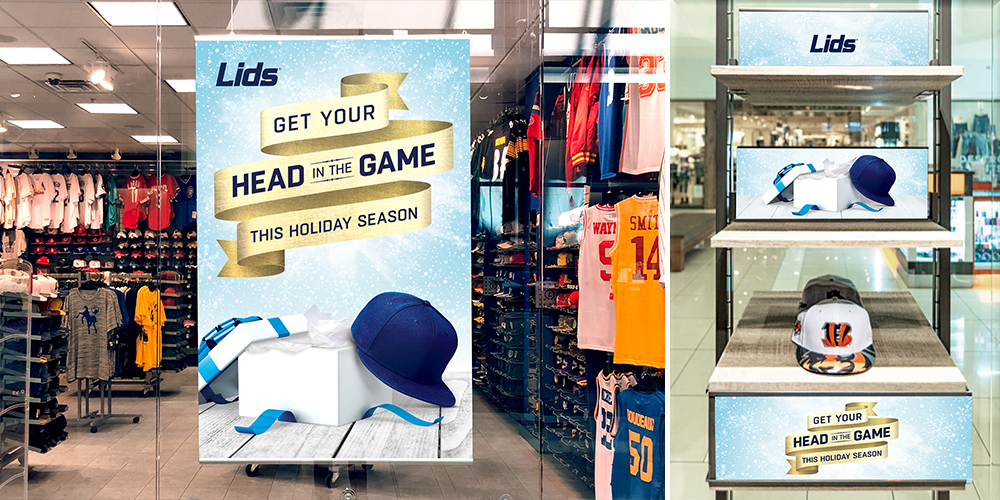The image depicts two sections within a sports merchandise store, intricately detailed to capture the festive retail atmosphere. The left two-thirds of the image showcase an interior view of the store from behind a glass pane, which is adorned with a sign that reads, "LIDS. Get Your Head in the Game this holiday season" in navy lettering. This sign features a golden ribbon and an illustration of an open white package with a blue ribbon, revealing a blue ball cap. The store behind the glass is vibrantly stocked with various sports paraphernalia, including t-shirts, jerseys, and ball caps bearing different logos and colors.

On the right third of the image, a set of retail shelves is displayed. The top shelf bears the word "LIDS" in navy, set against a blue and white snowy backdrop. Below this, the middle shelf replicates the sign from the left image, featuring the open present with the blue cap. The bottom shelf showcases two ball caps, each white with distinctive orange and black logos associated with the Cincinnati Bengals; one cap displays the team's "B" logo and the other features a tiger motif on the visor. Beneath this shelf is another instance of the "Get Your Head in the Game this holiday season" banner, reinforcing the festive retail theme.

Overall, the shared elements and repeated imagery between the two sections emphasize the store's branding and holiday promotional campaign, creating a cohesive and inviting shopping experience.